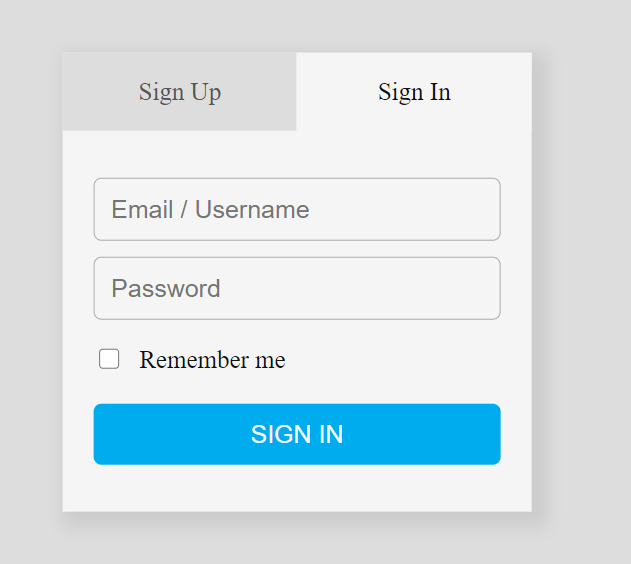The image captures a section of a website showcasing a user authentication interface. The background for this section is a gray square, featuring another white square box centrally placed within it. In the upper left corner of the white box are two tabs. The first tab on the left, which is not selected, is gray and labeled "Sign Up" in black text. Adjacent to it, the second tab is white, indicating it is the active selection, and bears the label "Sign In" in black text.

Below the tabs, the active sign-in form is displayed. The form consists of two gray-colored input boxes. The first input box is labeled "Email / Username," and the second is labeled "Password." Beneath these input fields is a white-background checkbox labeled "Remember Me" to its right. Further down, there is a prominent blue button inscribed with "Sign In" in white text, completing the sign-in section.